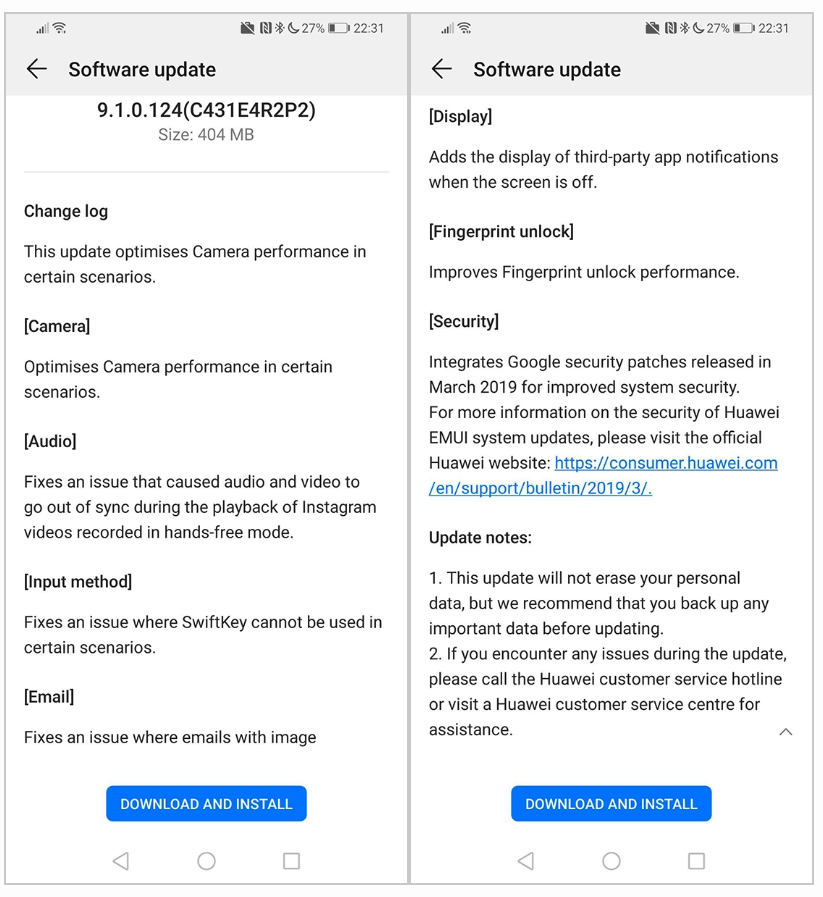This image displays two side-by-side screenshots from an Android device, highlighting a detailed software update notification.

**Left Screenshot:**
The left screenshot is from the 'Software Update' page, identifiable by the arrow at the top-left corner. The update is version 9.1.0.124 (C431E4R2P2), with a file size of 404 MB. The update features several categories:
- **Change Log:** Optimizes camera performance in certain scenarios.
- **Camera:** Enhances camera performance.
- **Audio:** Fixes an issue causing audio and video to go out of sync during Instagram video playback in hands-free mode.
- **Input Mode:** Resolves an issue where SwiftKey cannot be used in certain scenarios.
- **Email:** Corrects a problem with emails containing images.
A blue button labeled "Download and Install" is positioned at the bottom center.

**Right Screenshot:**
The right screenshot continues detailing the update:
- **Display:** Adds third-party app notifications display when the screen is off.
- **Fingerprint Unlock:** Improves the performance of fingerprint unlocking.
- **Security:** Integrates Google's security patches from March 2019 for enhanced system security. It also provides a link to the Huawei website for more information.
- **Update Notes:** 
   1. The update won’t erase personal data but recommends backing up important data.
   2. Contact Huawei customer service for issues encountered during the update, with details on the hotline number and service center locations.
This screen similarly has a blue "Download and Install" button at the bottom.

These screenshots provide a comprehensive overview of the software update's features and its importance for performance enhancements and security.